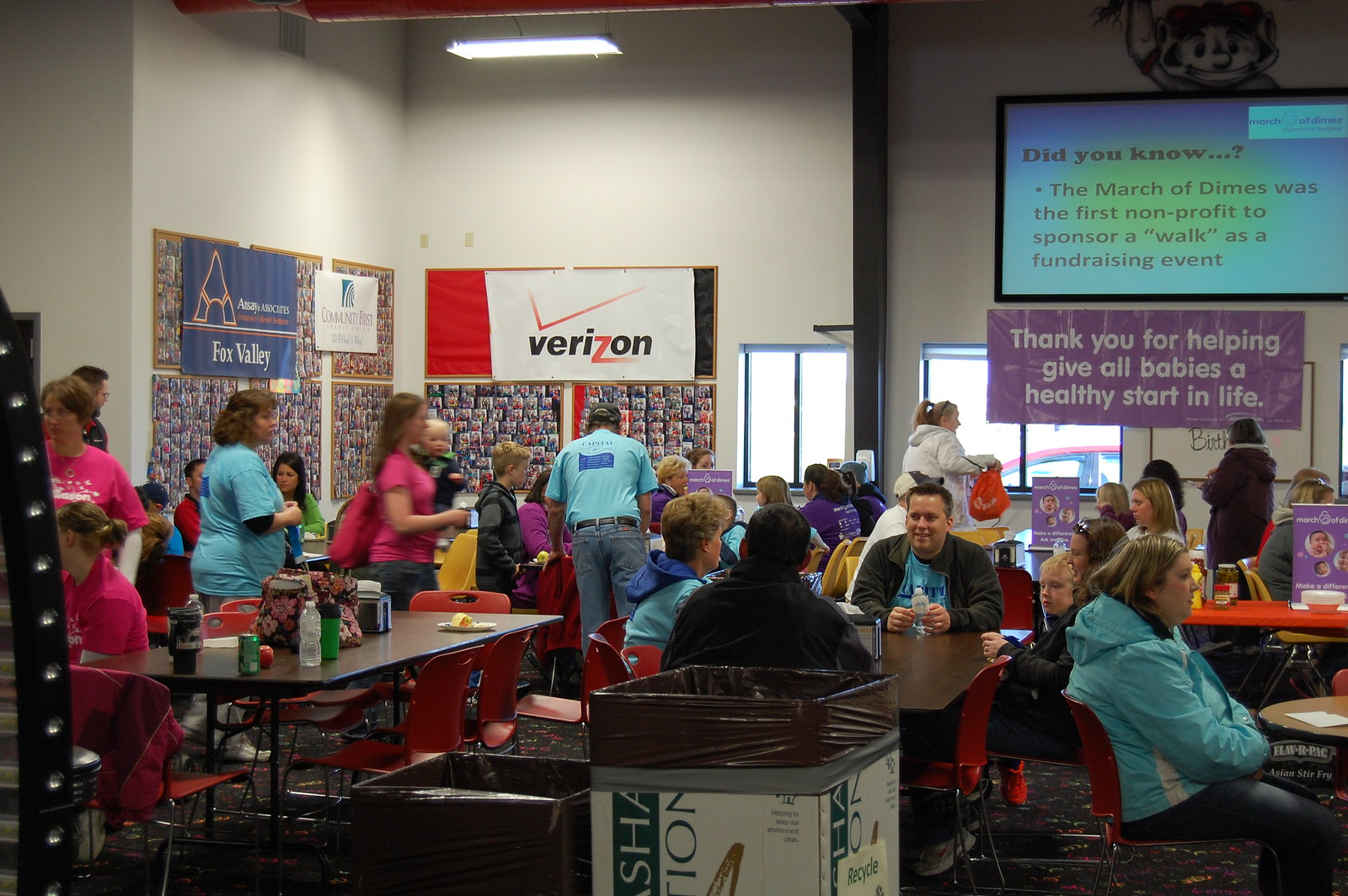This image depicts a large, horizontal rectangular space that appears to function as an employee cafeteria within a commercial building, possibly part of a hospital or corporate setting given the various contextual clues. The room is bustling with activity, with numerous people seated at tables and others standing and mingling. The tables accompany orange chairs, adding a splash of color to the otherwise white-walled environment. 

On one wall, there are several posters from different organizations, including Fox Valley, Community First, and Verizon. Prominently among these is a banner from the March of Dimes, expressing gratitude with the message, "Thank you for helping give all babies a healthy start in life." Above this banner, a large TV screen displays an informative statement noting that the March of Dimes was the first nonprofit to sponsor a walk as a fundraising event. This suggests that the gathering might be a fundraising event or a celebration of some kind.

The space also features practical amenities like vending machines and garbage cans, one of which is designated for recycling. Notably, there are workers or organizers in blue, pink, and purple shirts, indicating roles or affiliations, possibly related to the event or the organizations represented. The scene is lively, with an evident sense of community engagement and appreciation for the contributions made towards the cause, as indicated by the visible signage and bustling social interactions.